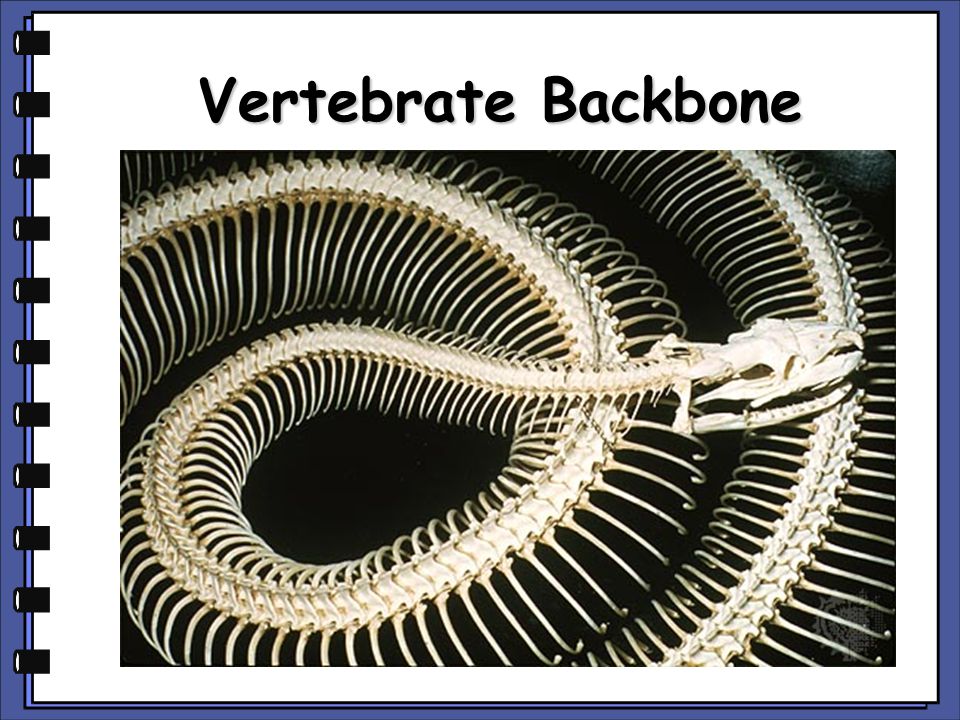The image titled "Vertebrate Backbone" features a highly detailed model of a snake’s skeleton against a contrasting dark background. At the top of the image, in bold dark letters, the title "Vertebrate Backbone" is prominently displayed over a white section. The dark blue outer border frames this central area, giving the impression of a page from an animated notebook or scrapbook. To the left side of the page, there are black, cartoon-styled staples or binders, suggesting it's part of a larger presentation or book report.

The photograph itself captures the intricate details of the snake's skeletal structure, which is composed of numerous white or cream-colored vertebrae and ribs. The snake's skull is positioned on top of the coiled backbone and rib cages, creating a visually striking circular pattern that fills the entire photograph. The rib cages and the spine bend with a sinuous grace, almost resembling a slinky. This meticulously crafted model highlights the complexity of the snake’s anatomy, making it a fascinating subject to observe.